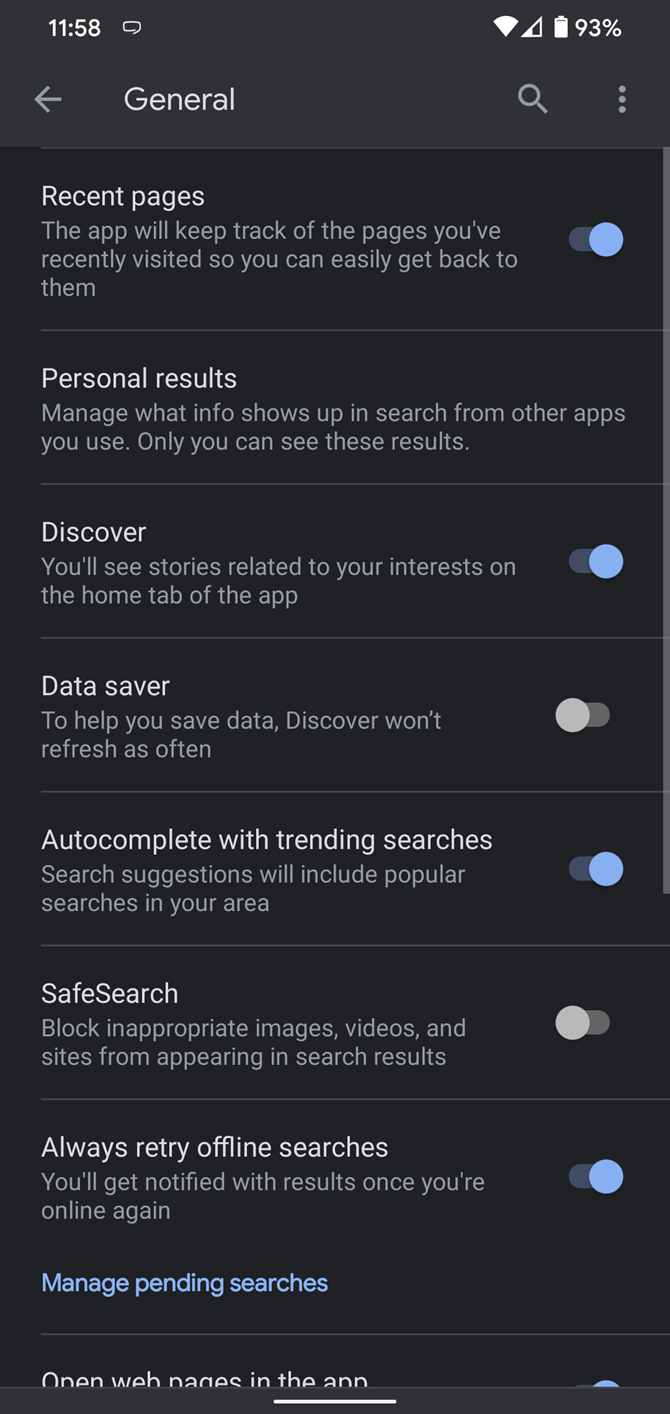The image appears to be a screenshot taken from a mobile phone, specifically displaying a settings menu from a web browser application. The background is entirely black. At the very top of the screen, the status bar displays the time as 11:58, with various icons including a fully charged battery at 93%. Below the status bar, a header labeled "General" is visible, accompanied by an arrow pointing to the left, a magnifying glass icon, and three vertical dots on the right side, likely indicating additional options or a menu.

In the main content area of the screen, a series of options with corresponding toggles are listed. On the left side of the screen, there are textual descriptions of each setting, while on the right side, there are slider switches to enable or disable each feature. The toggles are color-coded: when a setting is enabled, the toggle displays a blue circle on the far right, and when disabled, a gray circle appears on the left.

- The first setting, "Recent Pages," is turned on with a blue circle.
- "Personal Results" does not have a toggle switch.
- "Discover" is enabled, evidenced by the blue circle.
- "Data Saver" is turned off, displaying a gray circle.
- "Autocomplete with Trending Searches" is enabled, with a blue circle.
- "Safe Search" is turned off, shown by a gray circle.
- "Always Retry Offline Searches" is turned on, indicated by the blue circle.

Each setting listed provides customization options to enhance the browsing experience, with clear visual indicators for whether each feature is active or inactive.